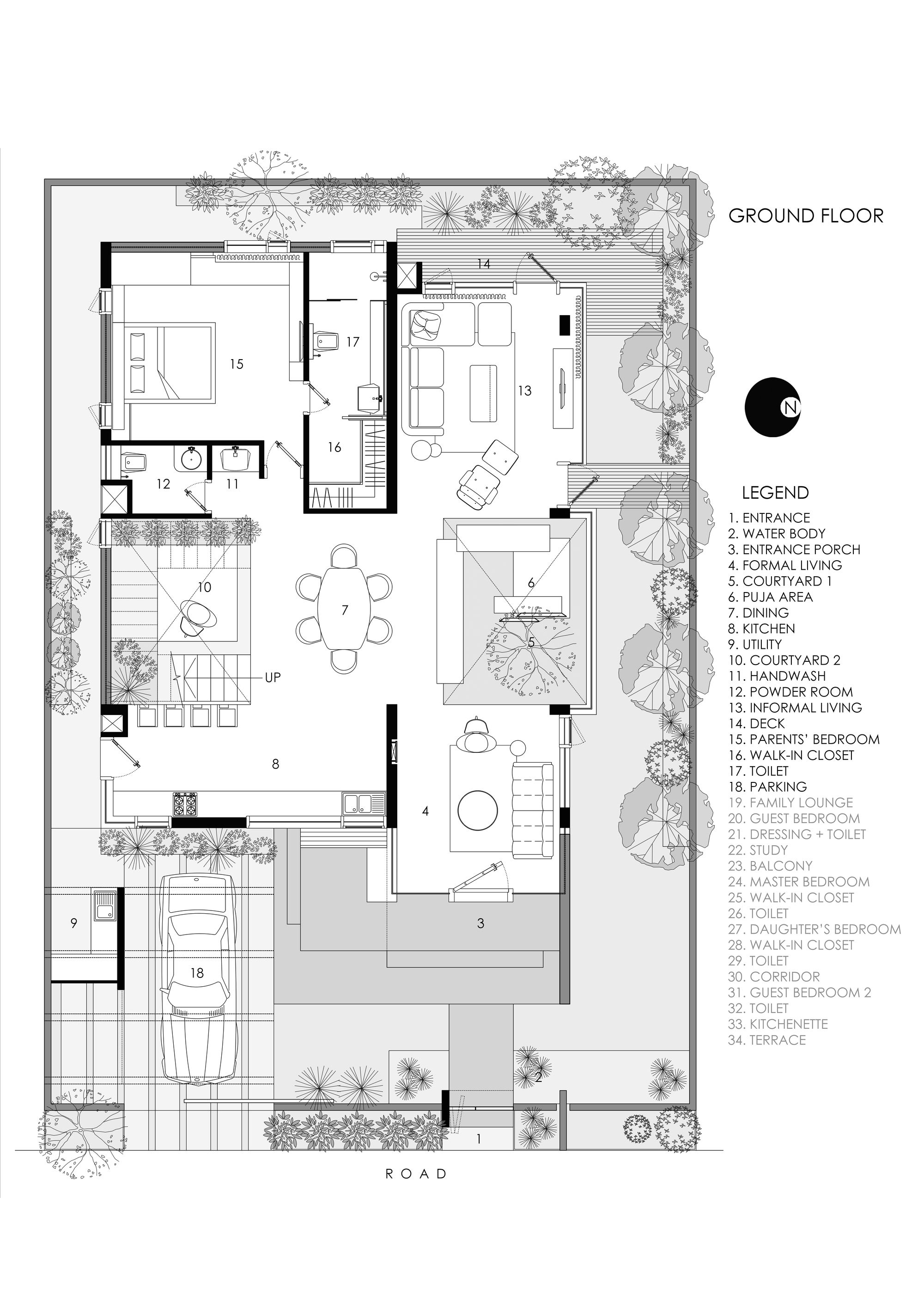This black-and-white, hand-drawn or computer-generated floor plan presents a detailed layout of the ground floor of a residential building. The image, viewed from an overhead perspective as if the roof had been removed, shows a variety of rooms and features within the house. The drawing includes areas such as the entrance, water body, entrance porch, formal living room, courtyard, puja area, dining room, kitchen, and utility area. Key furnishings and fixtures, like tables, sofas, beds, and major appliances, are visibly placed in respective rooms. Additionally, the plan features outdoor elements like a driveway with a car parked on the bottom left and surrounding clipart trees, with a road label at the bottom. On the top right corner, the image is labeled "Ground Floor." Adjacent to this label, a legend numbered from 1 to 34 lists various sections of the home, with entries such as guest bedroom and family lounge grayed out, indicating they're not present in this particular floor plan.